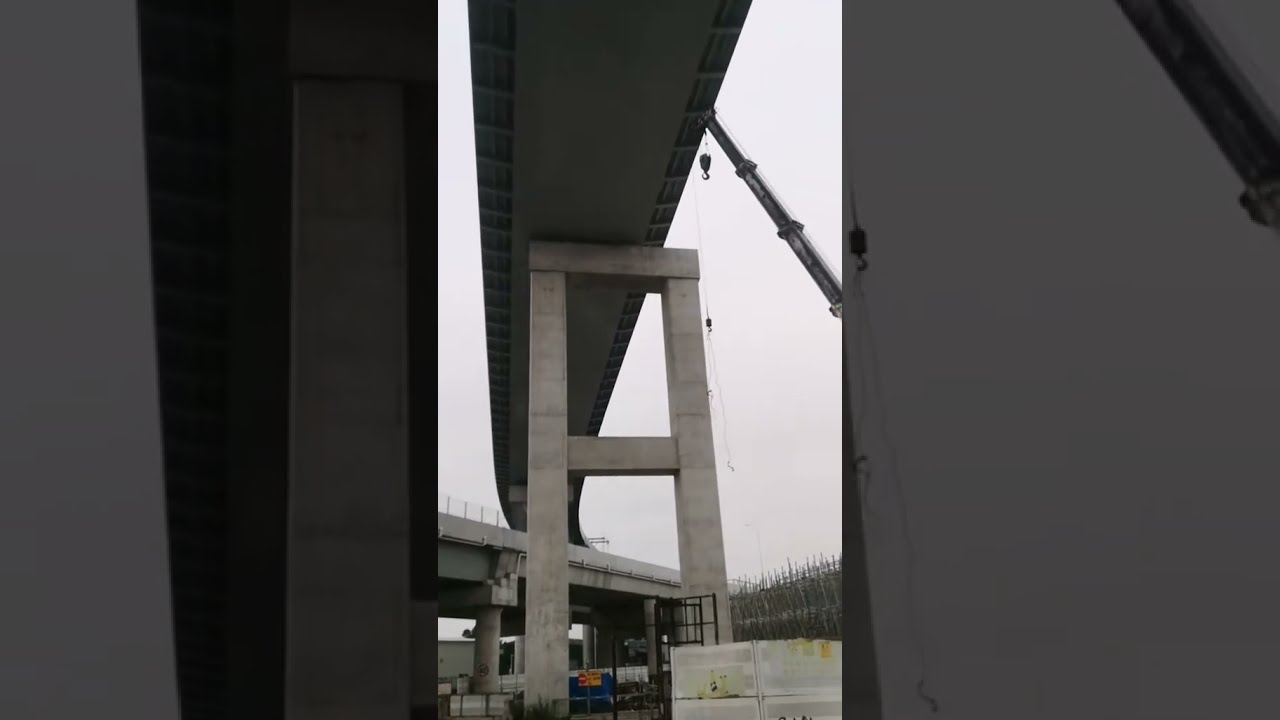The image captures the underside of an elevated overpass currently under construction. Dominating the foreground are large white cement stanchions that serve as the pillars, partially supporting the structure, with one stanchion noticeably extending only three-quarters of the way across the overpass. Visible from the left is a steel beam, while on the right, a crane arm extends diagonally across the image, with its hook suspended prominently at the top. The overpass itself has a dark gray underside, starkly contrasting the stanchions. Scattered around the construction site are various materials, including stone blocks and iron rods, indicating ongoing efforts to build the foundation and other sections. The sky above is overcast, casting a gloomy light over the scene. Additionally, the image features a blurred border that enlarges elements of the main picture to frame it subtly. In the background, another section of the freeway runs diagonally beneath the underpass, further emphasizing the complexity and scale of the construction.